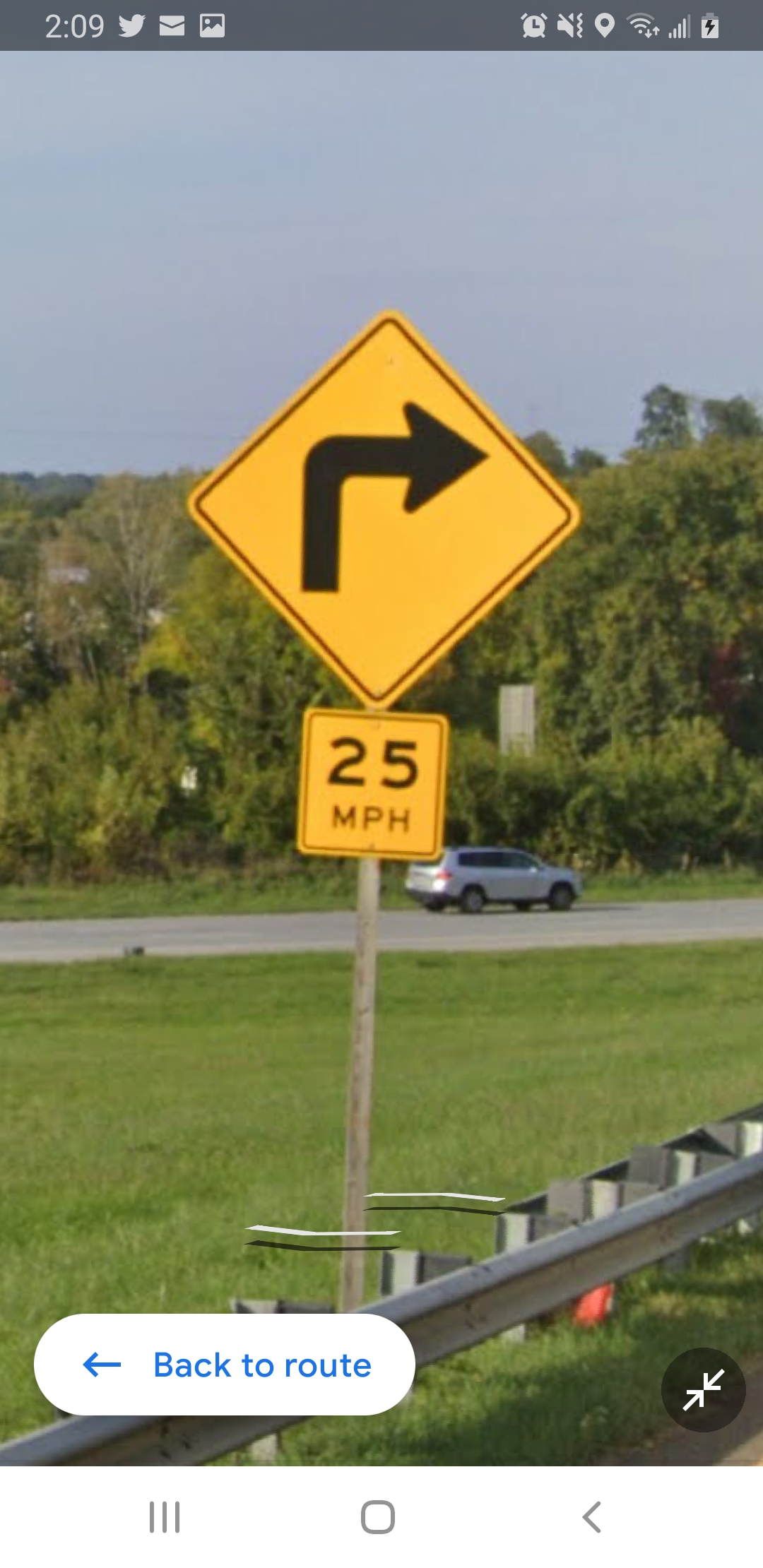This image is a screenshot captured from a smartphone or tablet device. At the top of the image, there is a grey status bar featuring white icons indicating the current time, an alarm clock, internet or data signal strength, and battery life. The primary content of the screenshot is a photograph taken within a map application, showcasing the side of a road. Prominently, there is a yellow road sign with a black arrow directing traffic to the right and a speed limit sign indicating 25 miles per hour. In the background, a silver car is visible traveling along the road. At the bottom of the screenshot, an infographic displays the text "Back to Route" accompanied by an arrow pointing to the left-hand side of the image.